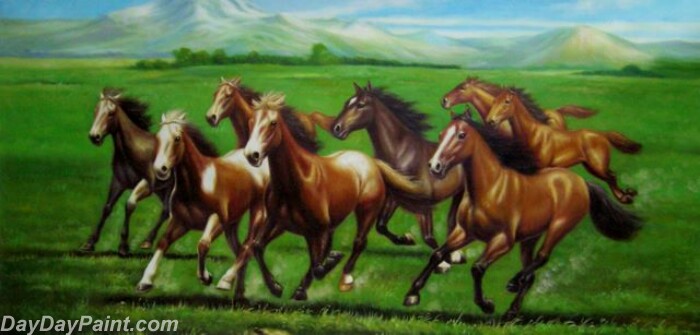This oil painting, executed on canvas, portrays a vivid and dynamic landscape scene. In the background, a blue sky is dotted with low-lying clouds, and majestic snow-capped mountains rise near the horizon. In front of these mountains stretches a lush, green field, flanked by a row of trees in the distance and another tree line towards the upper right side of the canvas. Dominating the foreground, eight wild horses, mostly chestnut brown with dark manes, are captured in mid-gallop, kicking up dirt to emphasize their movement. Among them, a palomino and a couple of horses with white patches on their backs stand out. The scene is imbued with a sense of freedom and vitality. In the bottom left corner, the artist's signature, "daydaypaint.com," is clearly visible in white font.